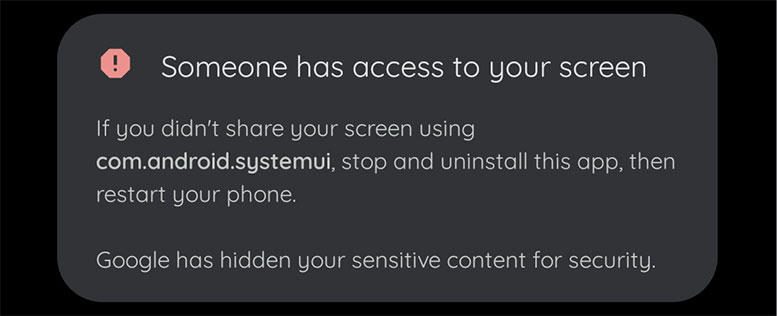A rectangular photo depicts a screen alert with a black background. Prominently, a large dark gray pop-up window with rounded corners is centered on the screen. 

In the top left corner of the pop-up, there's a red stop sign icon featuring a white exclamation point inside. Adjacent to this icon, bold white text declares, "Someone has access to your screen." 

Below this alert, smaller light gray text explains: "If you didn't share your screen using com.android.systemui, stop and uninstall this app, then restart your phone." 

At the bottom of the pop-up, it states, "Google has hidden your sensitive content for security."

This image represents a crucial system alert, warning the user about potential unauthorized screen access and advising immediate corrective actions.